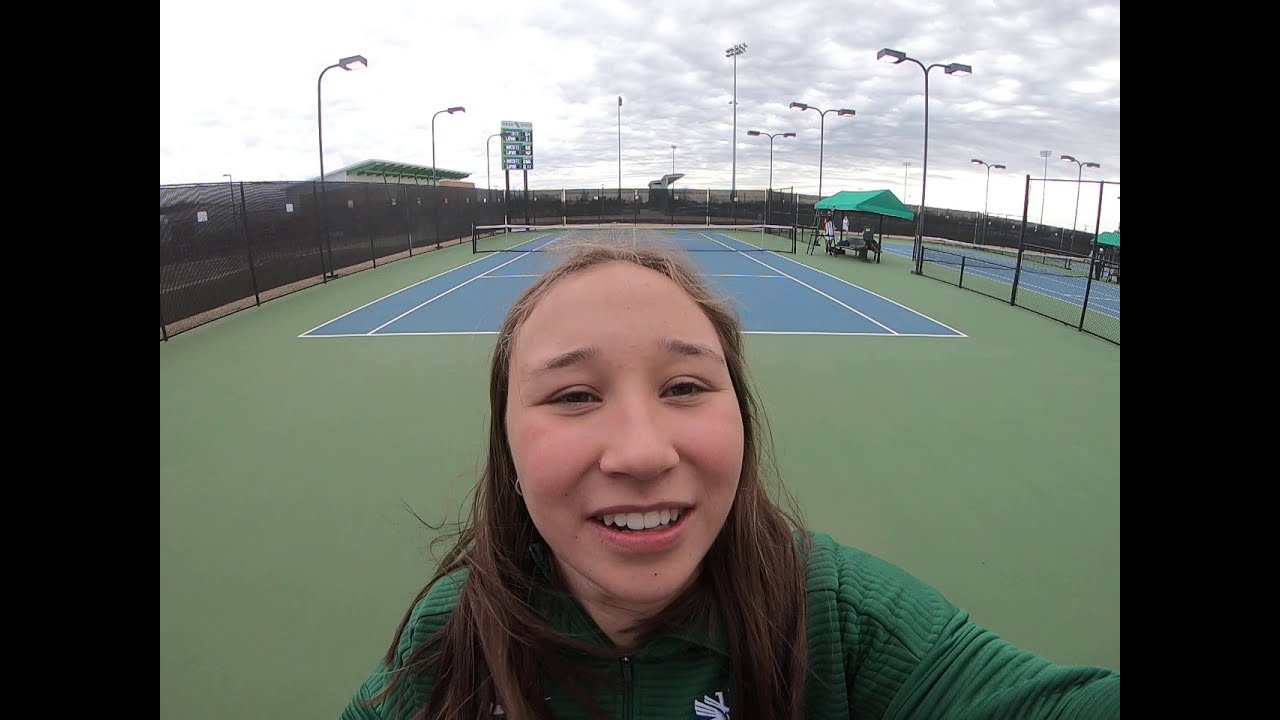A young girl, with a round face and a touch of redness in her cheeks, smiles directly at the camera, revealing her teeth and pink-colored lips. Her hazel eyes are slightly open, and her hair, appearing slightly wet, falls past her shoulders. She wears a long-sleeved green shirt. Behind her is a tennis court with a blue playing surface outlined in white lines, surrounded by a green surface. A net stretches across the center of the court, and a metal barrier circles the perimeter. There are poles with lights and a green and white scoreboard visible in the background. To the right of the girl, under a teal canopy, people are sitting and standing on benches. The overcast sky above is filled with gray and white clouds, suggesting recent rain. The setting is outdoors in the middle of a cloudy day on a tennis court.